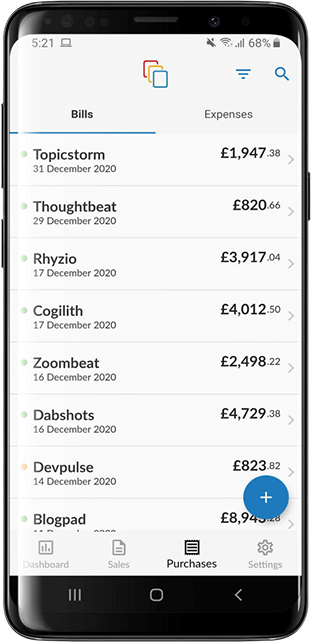A close-up image of a cell phone encased in a protective cover, displaying a meticulously organized screen. The device shows an application dedicated to managing bills and expenses, with the current screen focused on the "Bills" tab, highlighting a specific bill titled "Topic Storm" amounting to £1,947.38. The status bar at the top left indicates the time is 5:21, alongside a laptop icon suggesting connectivity. The upper right-hand corner shows the battery at 68%, full cell phone reception bars, full Wi-Fi signal strength, and the ringer set to silent mode. Just below the status bar, a logo of three stacked, transparent squares with colored edges is visible, presumably representing documents or pages within the application.